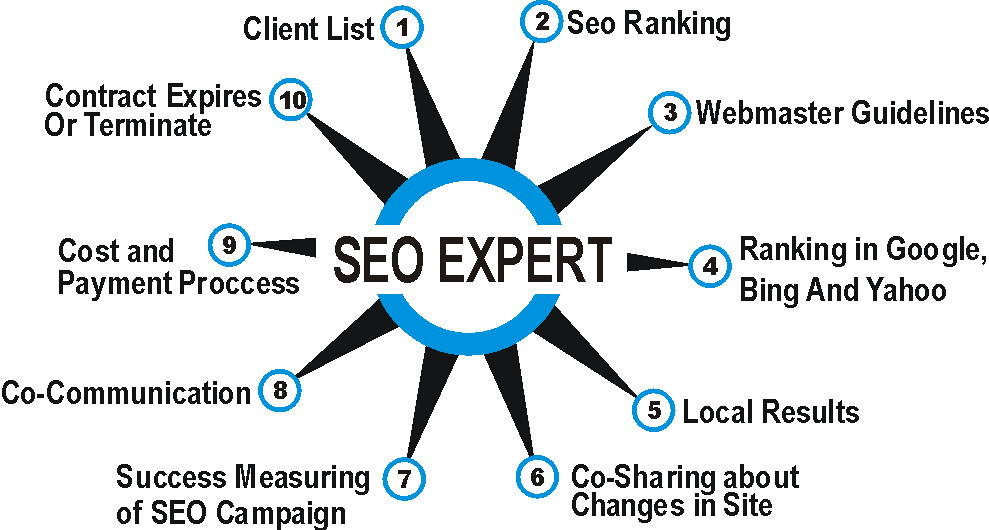The image is a detailed infographic meant to explain various aspects and offerings of an SEO strategy. At the center is the text "SEO Expert" printed in black, surrounded by a blue circle. Extending from the circle are ten starburst points, each labeled with numbers 1 through 10, and each containing relevant SEO topics. The points are designed in black and blue against a white background, visually resembling the rays of a sun or the hours on a clock. The topics listed at each point are: 1) Client List, 2) SEO Ranking, 3) Webmaster Guidelines, 4) Ranking in Google, Bing, and Yahoo, 5) Local Results, 6) Co-Sharing About Changes in Sites, 7) Success Measuring of SEO Campaign, 8) Co-Communication, 9) Cost and Payment Process, and 10) Contract Expiry or Termination. This infographic serves as a comprehensive guide or advertisement for understanding what an SEO expert entails and the services they provide.